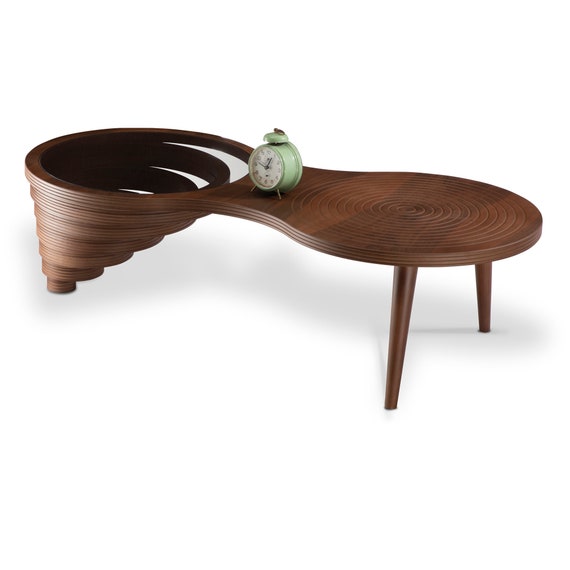This detailed image shows a uniquely designed wooden table with a rich brown color, set against a solid white background. The table has an unusual shape, resembling a figure-eight or a peanut, creating an intriguing visual appeal. On the left side, the table is supported by a hollow, spiral or cyclone-type structure that curls downward, giving it an almost floating appearance. On the right side, it rests on two sturdy legs and features intricate, concentric circular patterns on the surface, which are imprinted toward this side. An ancient-style, light green alarm clock is centrally placed on the table, adding a nostalgic touch to the scene. This clock, with its classic design, stands out against the dark wooden surface, enhancing the overall aesthetic of the image.